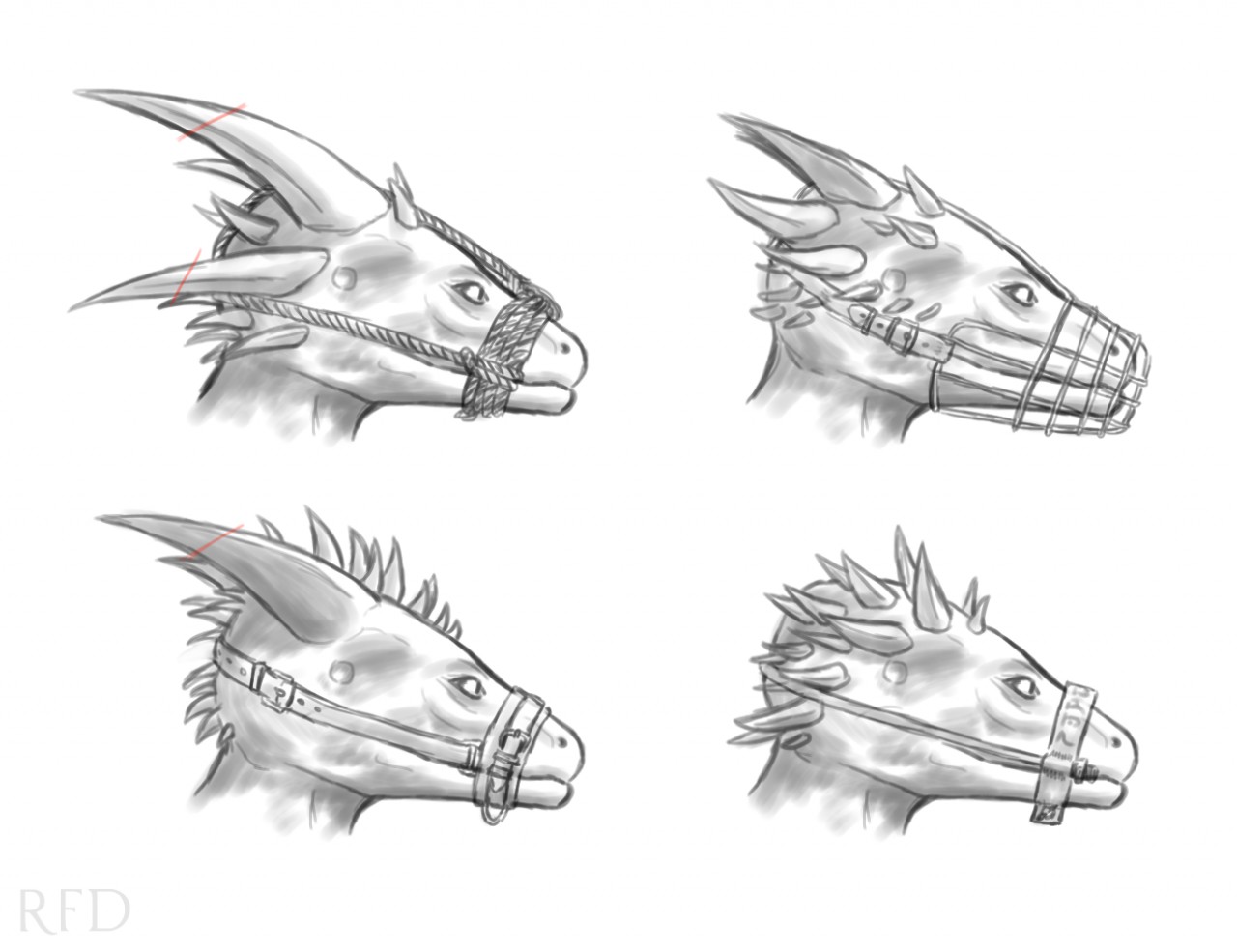This grayscale pencil drawing features four distinct representations of dragon-like creatures arranged in a perfect square grid, with each creature occupying one of the quadrants (upper left, upper right, lower left, and lower right). All four heads are depicted in profile against a monochromatic backdrop dominated by shades of black, white, and gray, showcasing intricate detailing and varying horn configurations.

In the upper left quadrant, the dragon’s head is adorned with large, prominent horns sprouting from the back. Its muzzle consists of a rope intricately tied around its mouth and cheeks, securing tightly behind its head. The upper right quadrant reveals a dragon with a collection of additional smaller horns on the sides of its head. This creature is bound by a cage-like muzzle with metal bands forming a crisscross pattern around its snout, fastened securely with straps.

The lower left quadrant showcases a dragon with a mohawk of small horns complemented by larger horns arching from the back. Its muzzle resembles a robust leather strap encircling its mouth, akin to a horse’s bridle. Finally, the dragon in the lower right quadrant displays an extensive array of medium-sized horns. Its muzzle, similar to a simple leather strap, features what appears to be writing or etchings and is secured with a screw mechanism.

Each dragon head is proportionally large and egg-shaped, narrower at the snout and broader at the base, exuding a prehistoric, dinosaur-like essence. The various muzzles signify an essential part of the artwork, emphasizing the unique restraint styles applied to each fantastical creature.